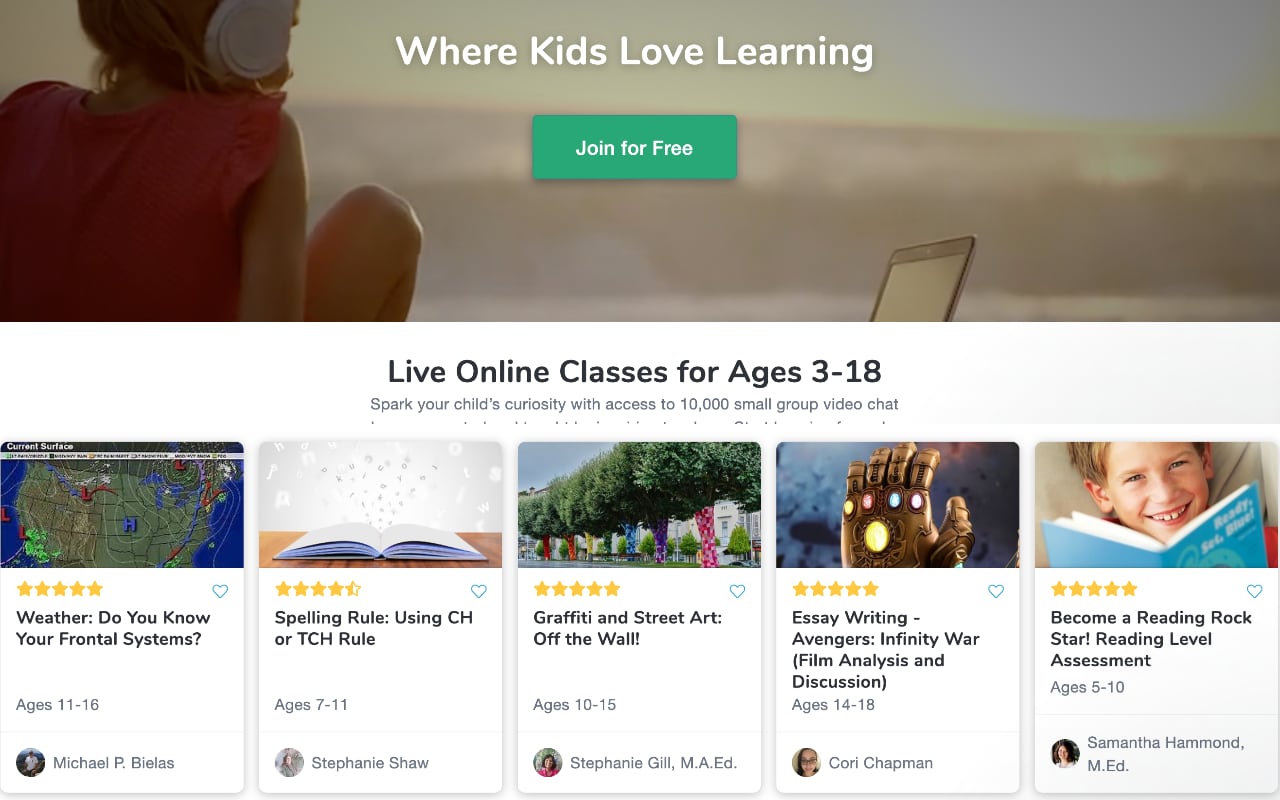This image is a screenshot from a website interface designed for a children's e-learning platform. The top third of the screenshot features a full-width banner image, bordered by a clean white margin. The central part of the banner showcases the tagline "Where Kids Love Learning" in a prominent white font. Directly below this slogan, a green rectangle is visible with the inviting call-to-action "Join For Free" written in white font.

On the left side of the banner image, there's the back view of a girl wearing a pink sleeveless shirt, partially revealing her right knee. Her head is mostly out of frame, with only the back of her head visible. Toward the right-bottom corner of the banner, the top edge of a laptop screen can be seen, albeit without any discernible content on its display. The background of this photo is blurred, hinting at what might be the silhouette of mountains under a gray sky.

Beneath the banner image, the background shifts to a crisp white. Here, bold black text announces, "Live Online Classes for Ages 3 to 18," followed by a smaller, non-bolded line of text stating, "Spark your child's curiosity with access to 10,000 small group video chat."

Below this section, a series of course listings are displayed in a horizontal format. Notably, each course features a rating system with gold stars, where one course has four and a half stars while the rest all have five stars. 

1. **"Weather: Do You Know Your Funnel Systems?"** - Accompanied by an image of a U.S. weather map reminiscent of those used in TV weather reports.
   
2. **"Spelling Rules: Using CH or TCH Rule"** - This course has four and a half gold stars. The corresponding image is a drawing of an open book with an array of white letters scattered in a playful background.

3. **"Graffiti and Street Art: Off the Wall"** - The image for this course includes trees, suggesting an urban art context.

4. **"Essay Writing Adventures: Infinity War (Film Analysis and Discussion)"** - A sci-fi themed image depicting the gloved hand of a character adorned with lights, likely referencing a popular film.

5. **"Become a Reading Rock Star: Reading Level"** - This course features a young white boy peeking over a book, embodying the target audience's age and curiosity.

This detailed description captures both the visual and textual elements of the website's screenshot, highlighting its educational focus and interactive course offerings for children aged 3 to 18.